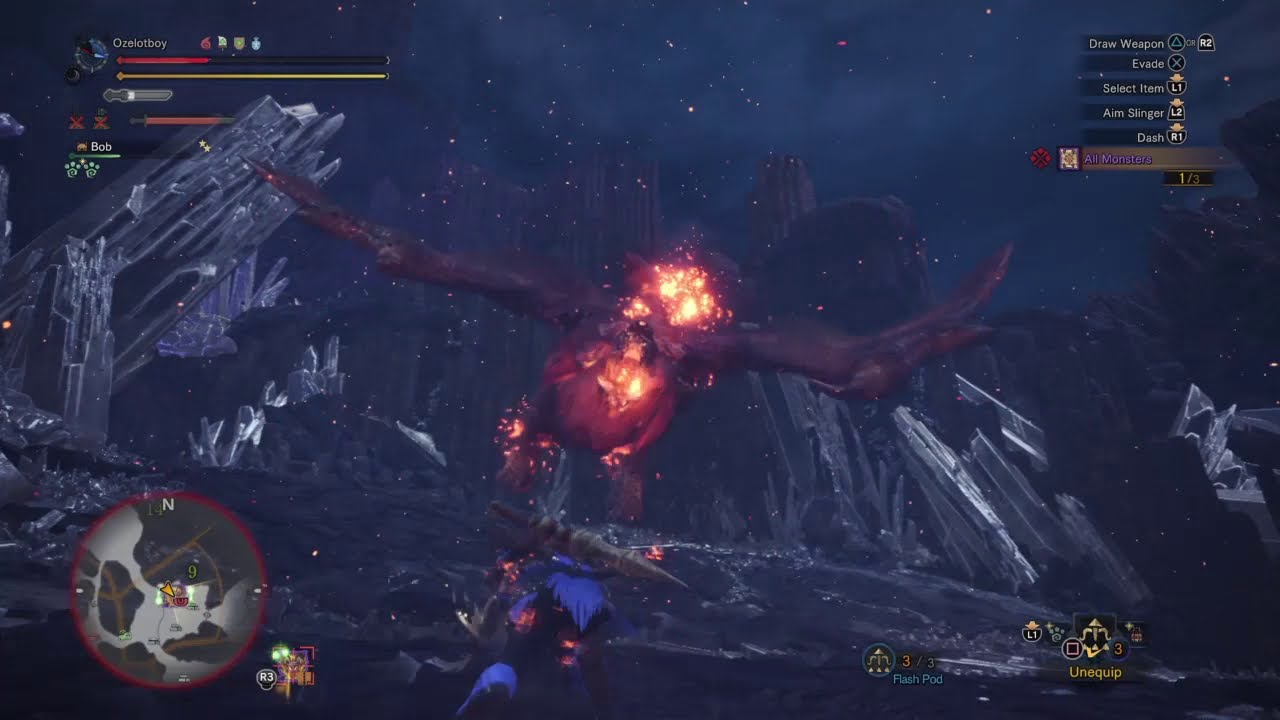The screenshot depicts an intense battle scene from a video game, set on a dark, alien landscape under a starlit night sky. Dominating the center of the image is a formidable dragon-like creature with flames emanating from its core, suggesting it is taking damage. The dragon has long, brown arms stretching from either side of its body, which is enveloped in an orange and yellow blaze. In the foreground, a character with blue hair and dark clothing stands with their back to the viewer, seemingly engaged in combat with the dragon.

The background features jagged, crystal-like structures rising high against the starry sky, contributing to the alien atmosphere. To the bottom left, a red circle displays an inset close-up of a platform with indistinct figures, potentially teammates or other characters. Nearby are various icons, including a radar. The bottom right corner houses an array of buttons and skill icons, labelled but unreadable.

The top left corner shows the boss's health bar alongside power levels and additional icons, providing critical information about the ongoing battle. In the top right corner, there's a scoreboard with names and numbers, further adding to the gaming data. The overall color palette includes black, gray, yellow, red, orange, green, blue, purple, and white, blending together to create a visually striking and intense scene characteristic of a video game experience.